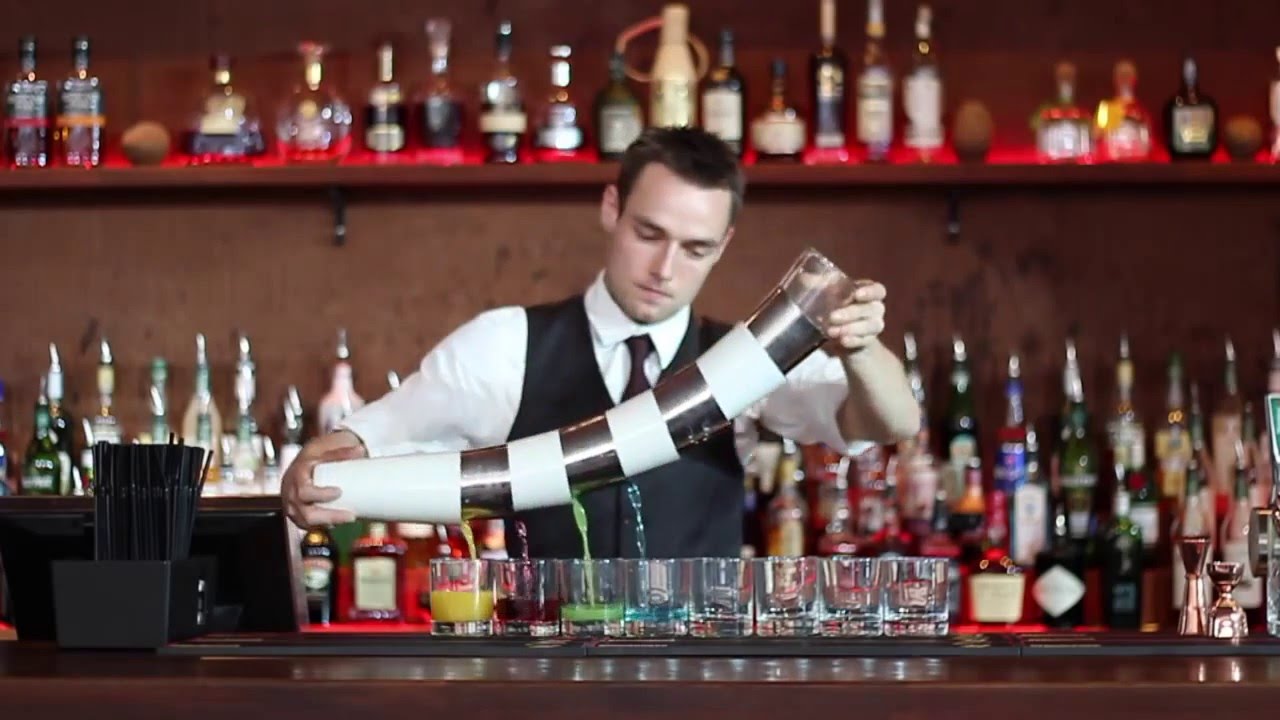The photo captures a mid-20s white male bartender with short, dark brown hair, positioned centrally behind a polished, brown wooden bar counter. He is dressed in a white collared shirt, a black waistcoat, and a black tie. The bartender’s hands are occupied with a stack of nested cups featuring a white and silver alternating pattern, presenting a curved column as he holds them together, seemingly preparing or performing a trick. Positioned in front of him on the counter are multiple shot glasses filled with drinks of various vibrant colors—yellow, dark red/brown, green, blue, and some that are clear or empty. To his left, a collection of straws is visible, suggesting readiness for cocktail mixing. Directly behind him, shelves adorned with an LED backlight emitting a red hue display an array of liquor bottles of varying sizes. To the right, possibly a tap or another piece of bar equipment peeks into view. The bartender is focused and concentrated on his task amidst the lively and colorful bar setting.